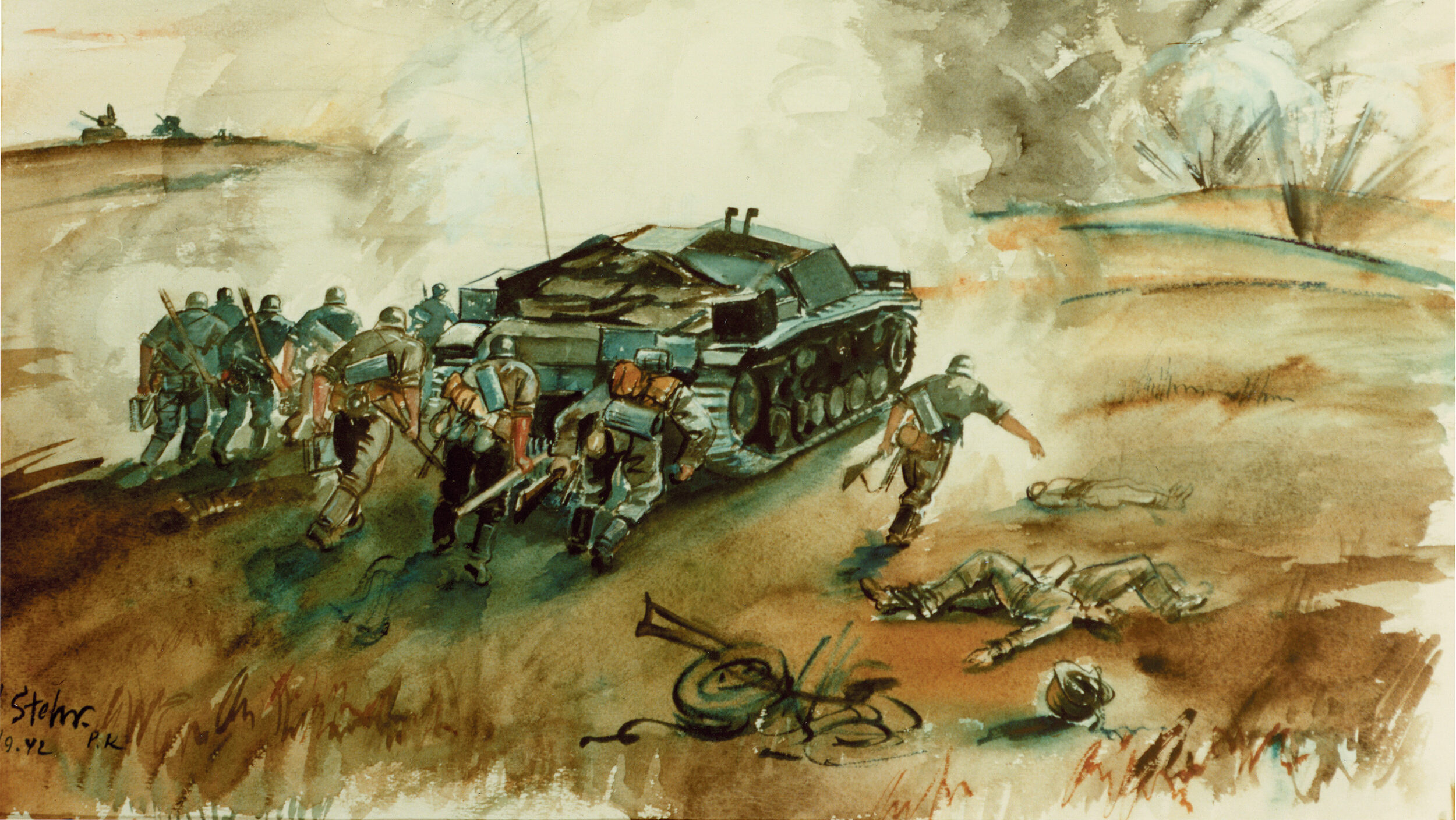This is a detailed, hand-painted watercolor illustration depicting a wartime battlefield scene. The overall color scheme is predominantly shades of brown and green, emphasizing the sense of desolation and muted atmosphere typical of war depictions. The landscape features rolling hills with areas of brown grass and sparse, dark-colored trees. The sky is a stark white, intermingled with clouds of gray smoke, indicative of recent explosions and ongoing conflict.

In the center of the image, a large greenish-gray tank, viewed from the rear, dominates the scene. It has distinctive metal panels, wheels, and tracks on each side. Marching behind the tank, around fifteen soldiers, clad in dark green-gray military uniforms with steel helmets, advance across the hilly terrain. Each soldier bears a rifle with a brown stock, and many carry additional gear such as black boots, belts, and brown backpacks.

Scattered throughout the foreground and middle ground are fallen soldiers, along with discarded items like dark tires and helmets. On the far left, additional tanks can be seen in the distant horizon, accentuating the expanse of the battlefield. There is a notable area near the upper left corner where smoke billows prominently, further underlining the turmoil of the scene.

In the lower left corner, the artist’s signature, potentially reading "ST EHR PK” and dated “94 L,” is visible, serving as a final touch to this evocative piece of war art.